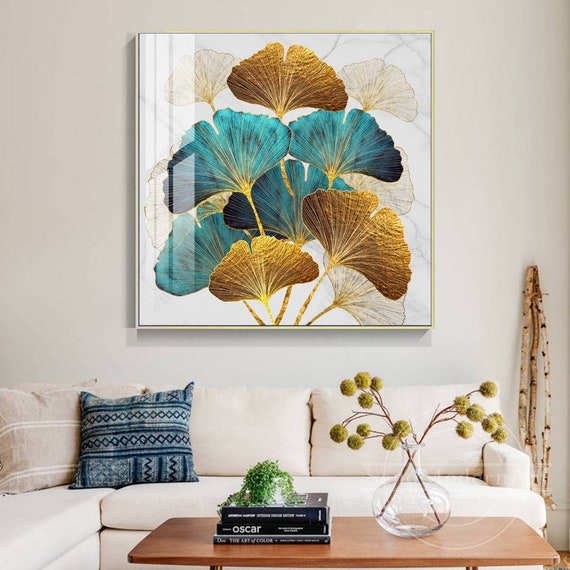This detailed photograph captures a meticulously staged living room, likely intended for a real estate listing. The focal point is a large square artwork mounted on the wall, showcasing vivid, pressed ginkgo leaves in an array of colors, including shiny gold, bright teal, and green, set against a white marble-like background and framed in tan.

Below the artwork, a cream-colored L-shaped sectional sofa is adorned with pillows, including a standout blue feature cushion. In front of the sofa, a wooden coffee table is neatly arranged with a stack of three black-spined coffee table books. To the left, there's a small potted plant with overflowing green leaves in a white pot. On the right side of the table, a clear glass vase holds decorative stems with soft, fuzzy green balls on top, alongside what appear to be bamboo sticks leaning against the sofa. 

The overall aesthetic of the room is tidy and neutral, with light or tan hues prevailing throughout the space, offering a warm and inviting atmosphere.